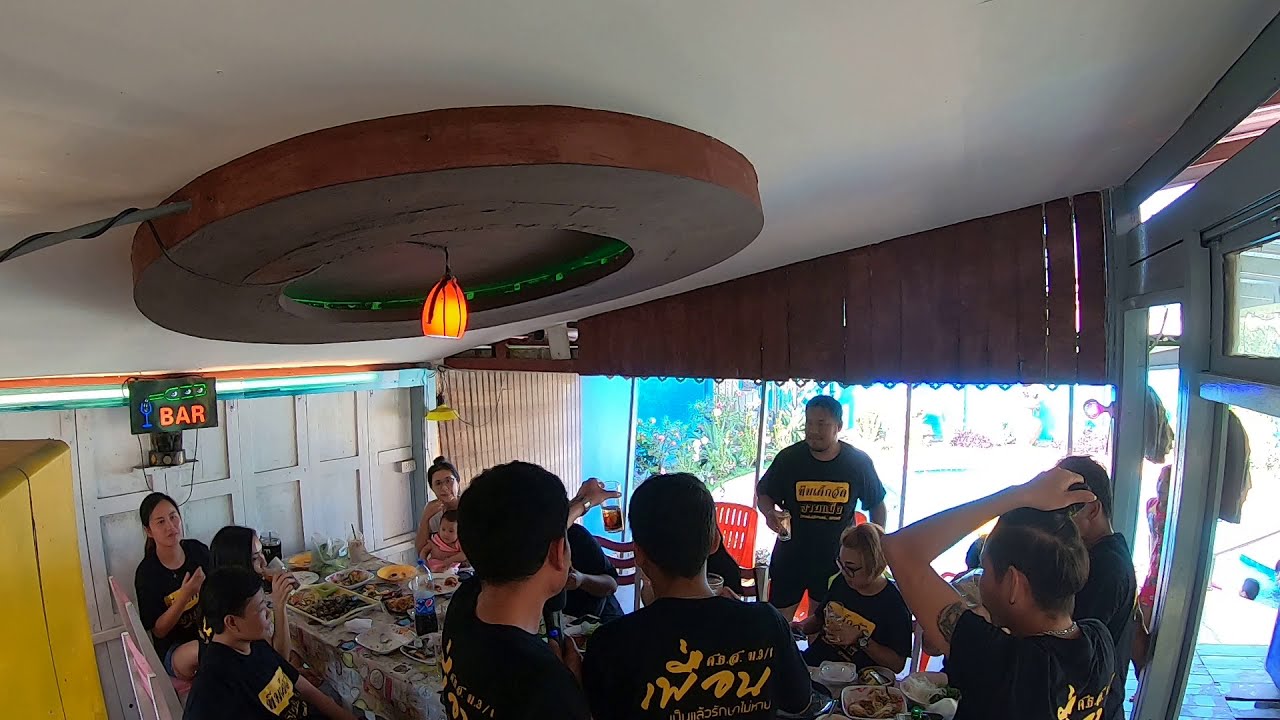Inside a cozy Thai restaurant, a group of about 11 young men and women, possibly in their 20s, are gathered around a long table filled with an assortment of Asian food and drinks. They're all dressed in matching black t-shirts emblazoned with a yellow logo and writing, which appears to be in Thai script. Positioned near the restaurant's door and a large window that overlooks a patio, the group enjoys their meal with some seated and others standing around the table. Prominently featured in the background is a neon sign that reads "bar" in bright orange letters, and a distinctive circular ceiling decoration with a light hanging from its center captures attention from above. One man, closest to the right, has his arm raised with his hand on his head, while another person holds up a glass in a toasting gesture.